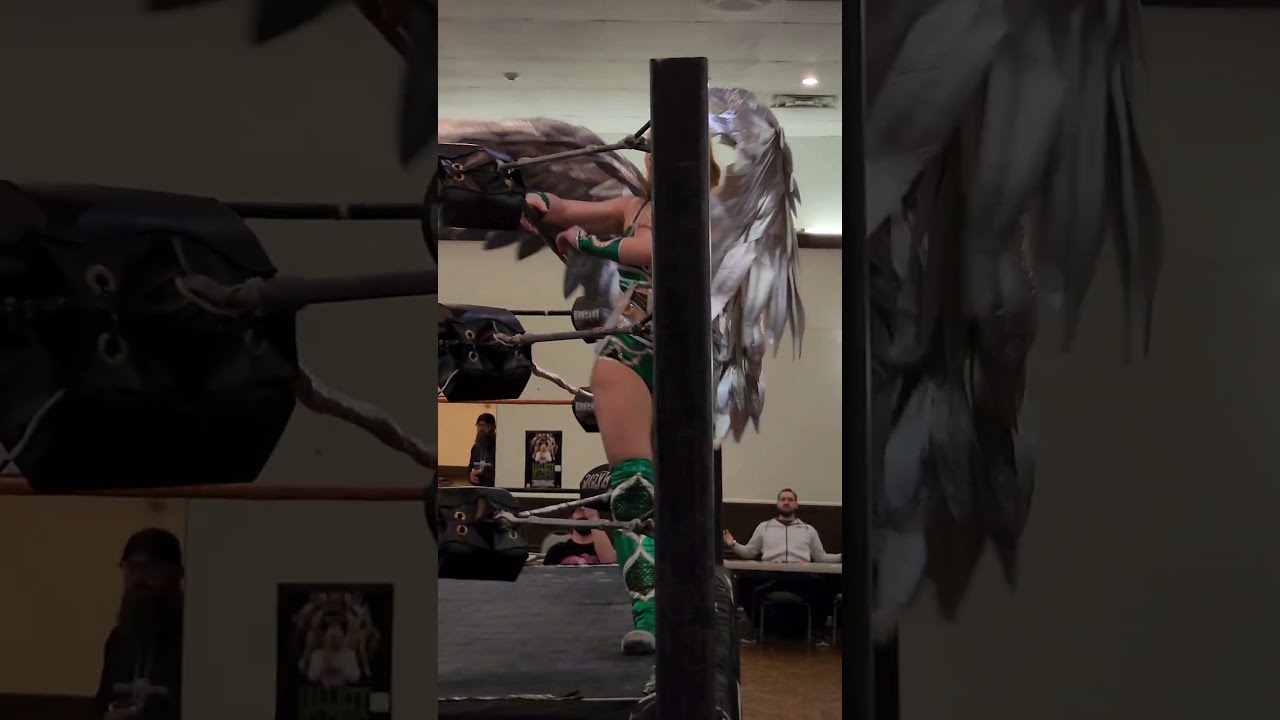The image is a composite photograph featuring three panels. The outer panels are zoomed-in, darker-toned sections of the same central image, arranged in a landscape orientation. The central panel, in portrait orientation, shows a wrestling ring with a gray floor and prominent corner posts and ropes. The main subject is a female wrestler, depicted in mid-action with one arm and leg visible from behind the post. She is dressed in knee-high green and black boots, a green and black bathing suit-style outfit with shoulder straps, and matching green, yellow, and black wristbands. Her head is adorned with a large, gray and white feathered headdress that cascades down to her knees, resembling angel wings.

The background features a sparsely populated room with a few spectators seated at small tables, giving the impression of a private event or practice session rather than a full match. One man in a white shirt is seated on the floor near a desk or counter, while another individual is visible near the left background, with pictures adorning the walls behind them. The photograph incorporates elements of both photo-realism and manga-style illustration, particularly noticeable in the superimposed manga female head with long, feathery hair on the right side of the wrestling ring post. The overall composition creates a dynamic and festive atmosphere, highlighting the theatrical nature of the wrestling event.